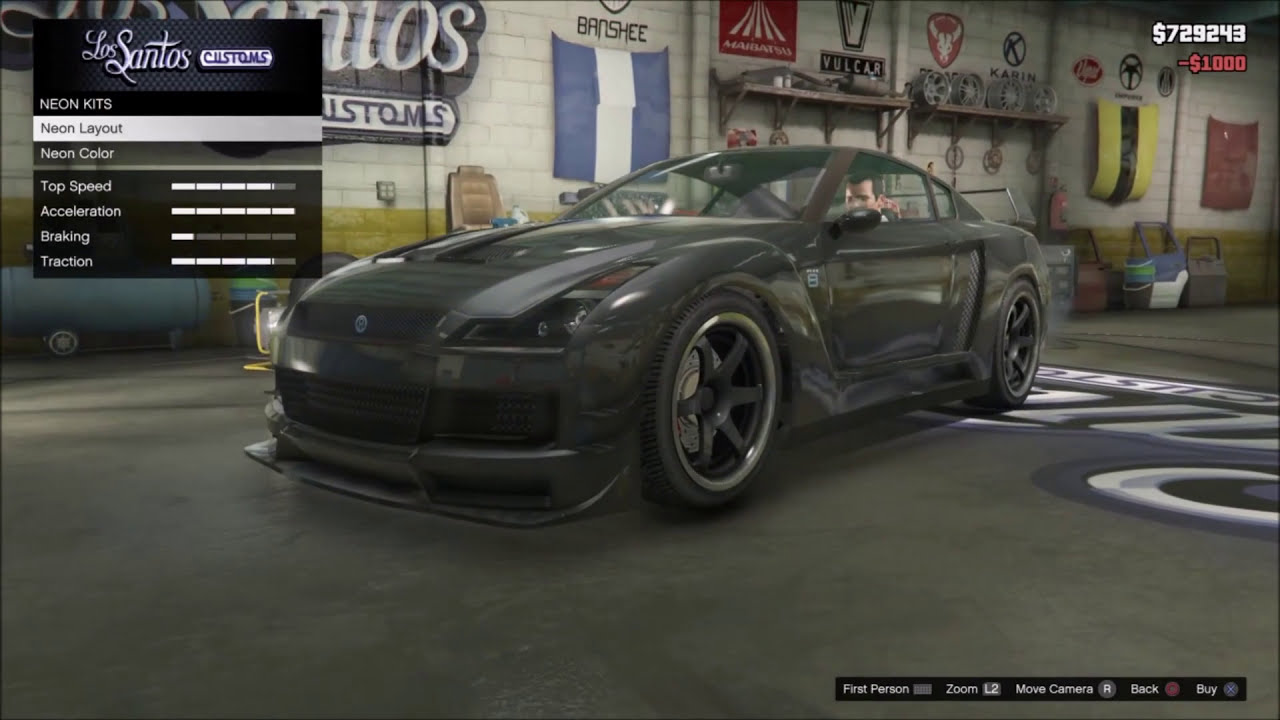The image is a detailed screenshot from the video game Grand Theft Auto 5. It features a sleek, dark charcoal gray sports coupe, named Bansky, parked inside a well-lit garage setting of Los Santos Customs. The car has a reflective sheen, large chrome rims, thin tires, and prominent vent detailing on the doors, alongside stylish curved angles on the hood. The garage floor is concrete, with a logo spray-painted on it, surrounded by a white brick wall with a thick yellow stripe at the bottom. The wall is adorned with various automotive parts like car hoods and rims, mounted on floating shelves.

To the left of the image, a game interface overlay displays options for customizing the vehicle, including neon kits, layout, color, as well as metrics for top speed (four bars), acceleration (five bars), braking (one bar), and traction (four bars). The top right corner shows the character’s total money as $729,243, with a red deduction of $1,000 for current modifications. Further, the bottom right corner of the interface allows for different camera views and actions such as first person, zoom, move camera, back, and buy. In the driver's seat of the car, a character with dark brown hair is visible, underscoring this dynamic customization scene.